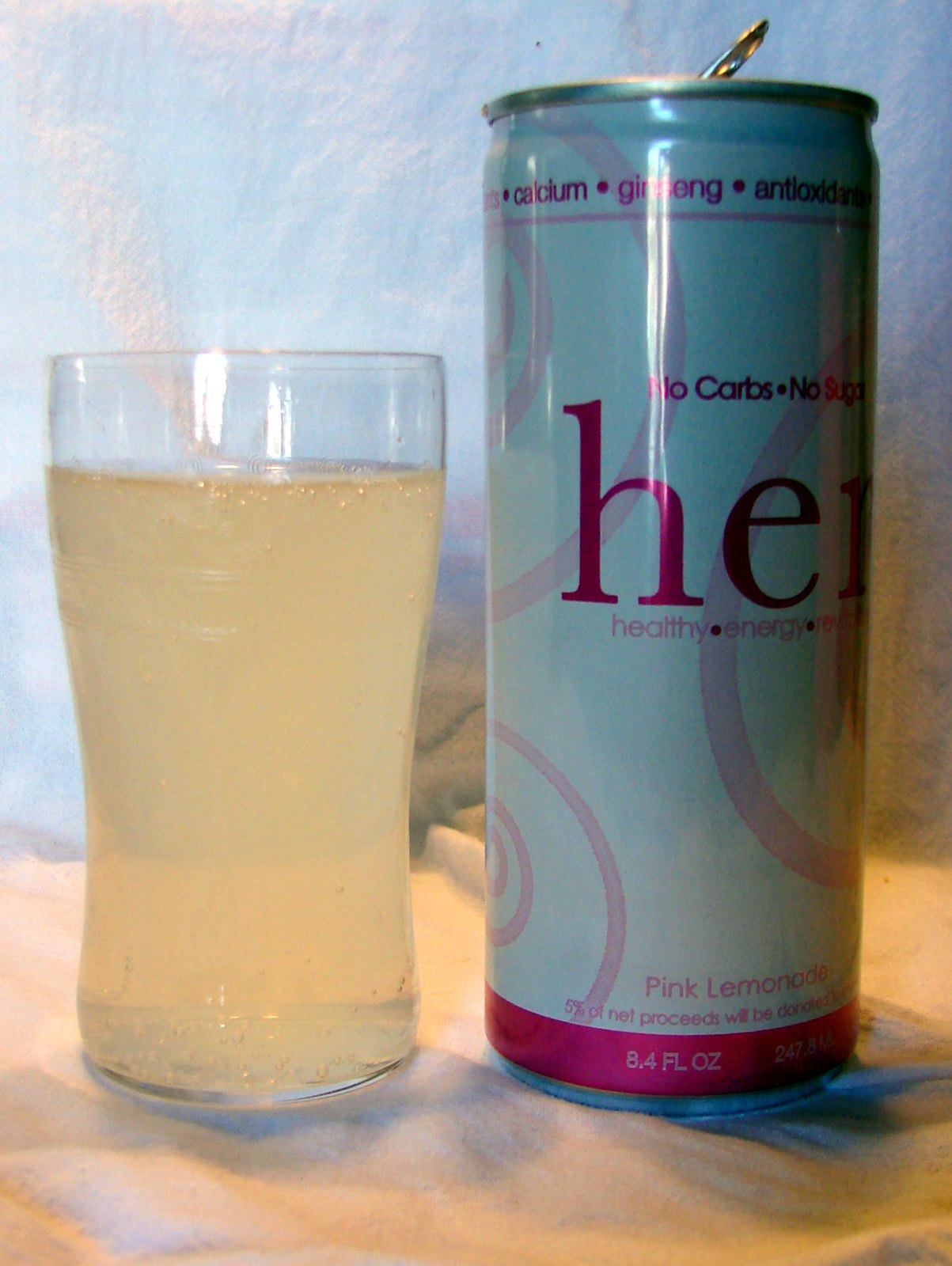The image showcases a photograph of a beverage can labeled "HER," which stands for "Healthy Energy." The can prominently displays various health claims such as "calcium," "ginseng," "antioxidants," "no carbs," and "no sugar." Additional text notes that "5% of proceeds will be donated." The flavor indicated is "Pink Lemonade," and the can has a capacity of 8.4 fluid ounces. 

The can itself is predominantly white with pink lettering and lighter pink accents. Notably, the section where "8.4 OZ" is printed shifts to a bright pink hue. Next to the can, there is a clear, curved glass containing a pale yellow liquid, presumably the beverage from the can. 

The background consists of a white cloth, and the overall photograph appears to be taken indoors with a slight blur.